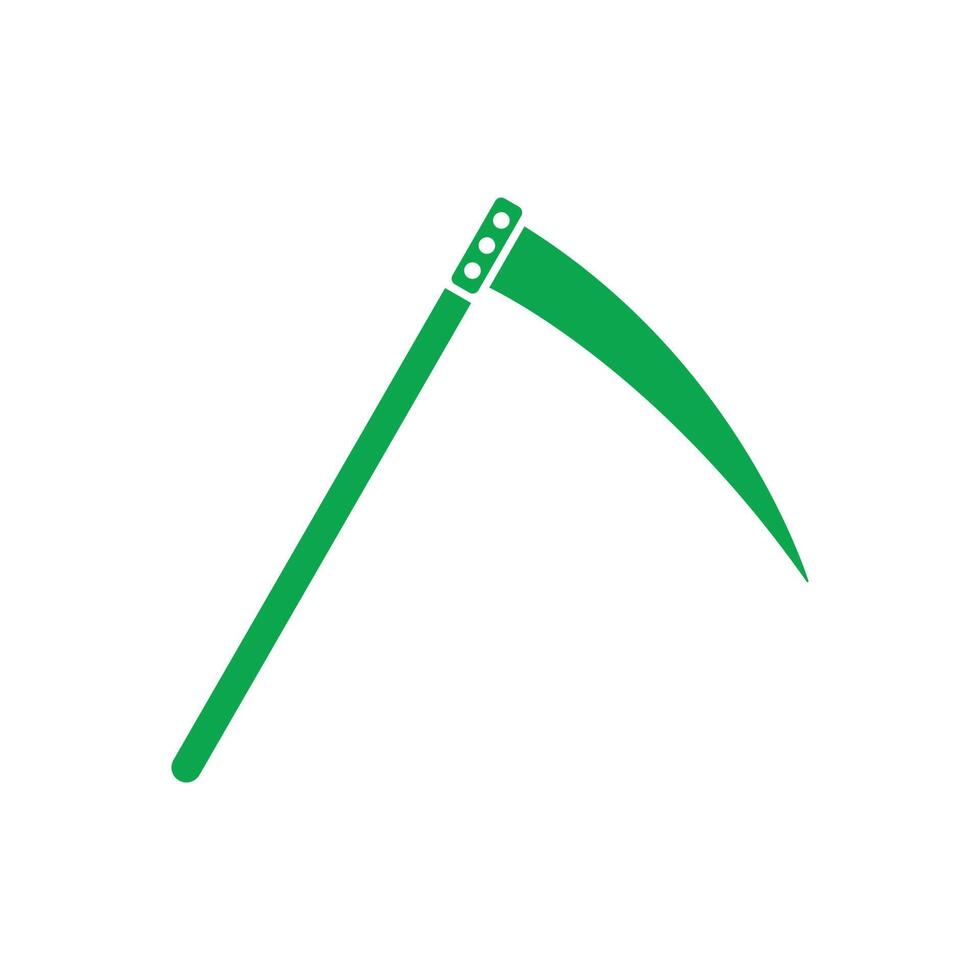This image features a simple, cartoonish depiction of a scythe or Grim Reaper's weapon, rendered in a bright forest green. Set against a clean, white background, the icon stands out distinctly. The scythe is approximately two inches high and consists of three main parts. First, the handle extends diagonally from the bottom left to the top right, resembling a rounded-bottom, flat-top green stick. The handle is positioned at a two-o'clock angle. At the top of the handle, a smaller section with three white dots appears, suggesting how the blade is attached. The blade itself is solid green and curves downward in a semi-circular arc, pointing towards the five-o'clock position. The overall design is reminiscent of a large emoji or clip art, characterized by its simple and clean lines.